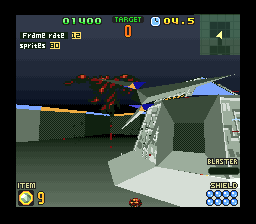This image is a highly detailed screenshot from a video game, capturing an intricate, silver and gray spaceship-like structure. The structure is adorned with numerous buttons and panels, enhancing its futuristic appearance. In the top right corner of the screen, a directional map is visible, aiding in navigation. At the bottom, icons labeled "SHIELD" and "BLASTER" can be seen, indicating available gameplay features. The player's score is displayed as 01400, with the target marked as 0, and a countdown timer showing 04.5 seconds remaining.